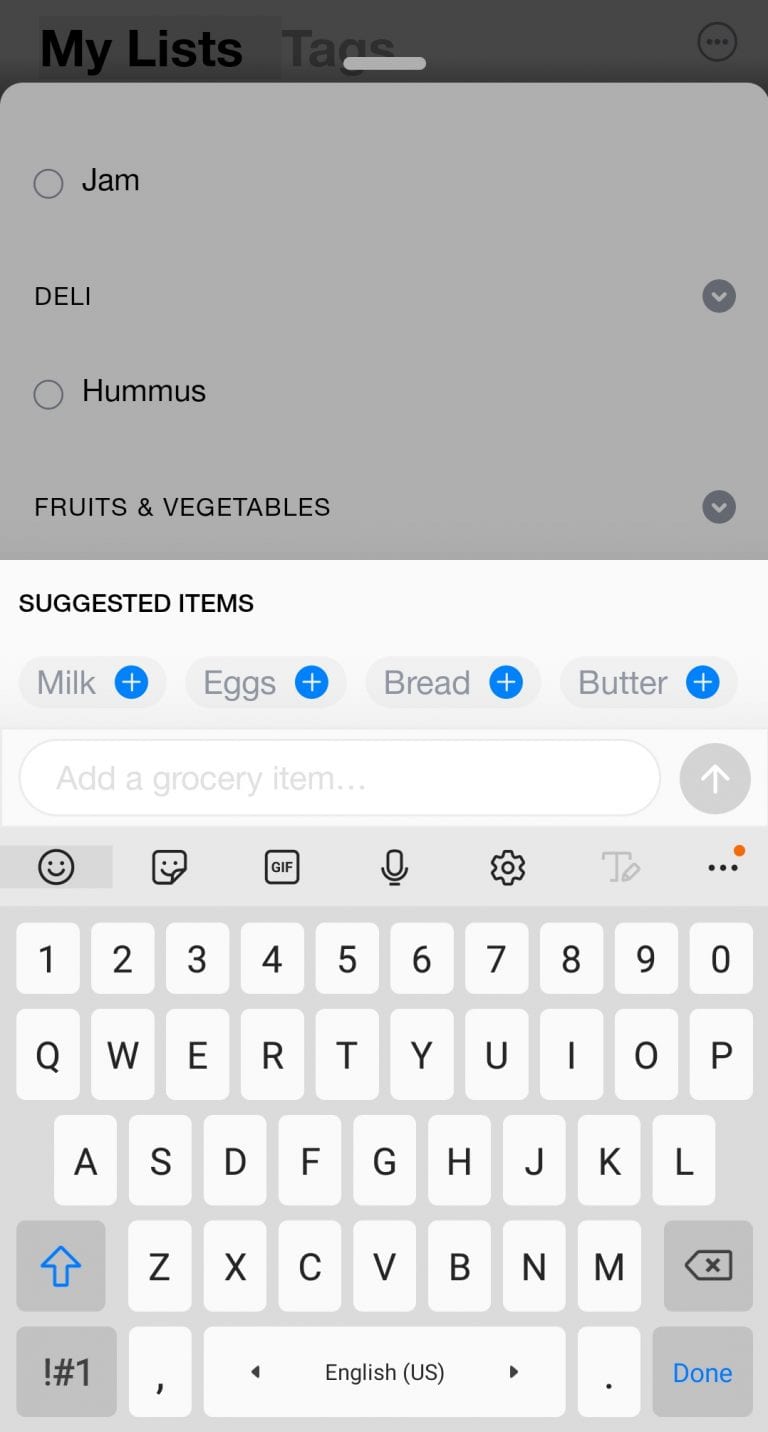The image displays a user interface with several distinct sections and buttons. At the top, there is a black box featuring a thin gray line. Below this, a gray box contains several items: a small circle labeled "jam" with the word "deli" next to it, followed by a black circle with a check mark on the right. Another small circle labeled "hummus," accompanied by the words "fruits and vegetables" and another black circle with a check mark, is also visible.

Further down, a light blue box reads "Suggested Items" and includes buttons for "milk," "eggs," "bread," and "butter," each accompanied by a blue circle with a plus sign. 

Next, a white search bar is displayed with a gray circle featuring an upward-facing arrow.

Below the search bar, a gray box is populated with icons for a smiley face, a small square, a GIF, a microphone, settings, a large "T," a smaller square beside it, and three dots with a red circle over them.

The keyboard interface includes a blue up arrow, followed by buttons for an exclamation point, a hashtag, and the number one. In the center of the keyboard, the word "English" is displayed with arrows pointing left and right. Finally, a gray button labeled "Done" in blue is situated at the bottom.